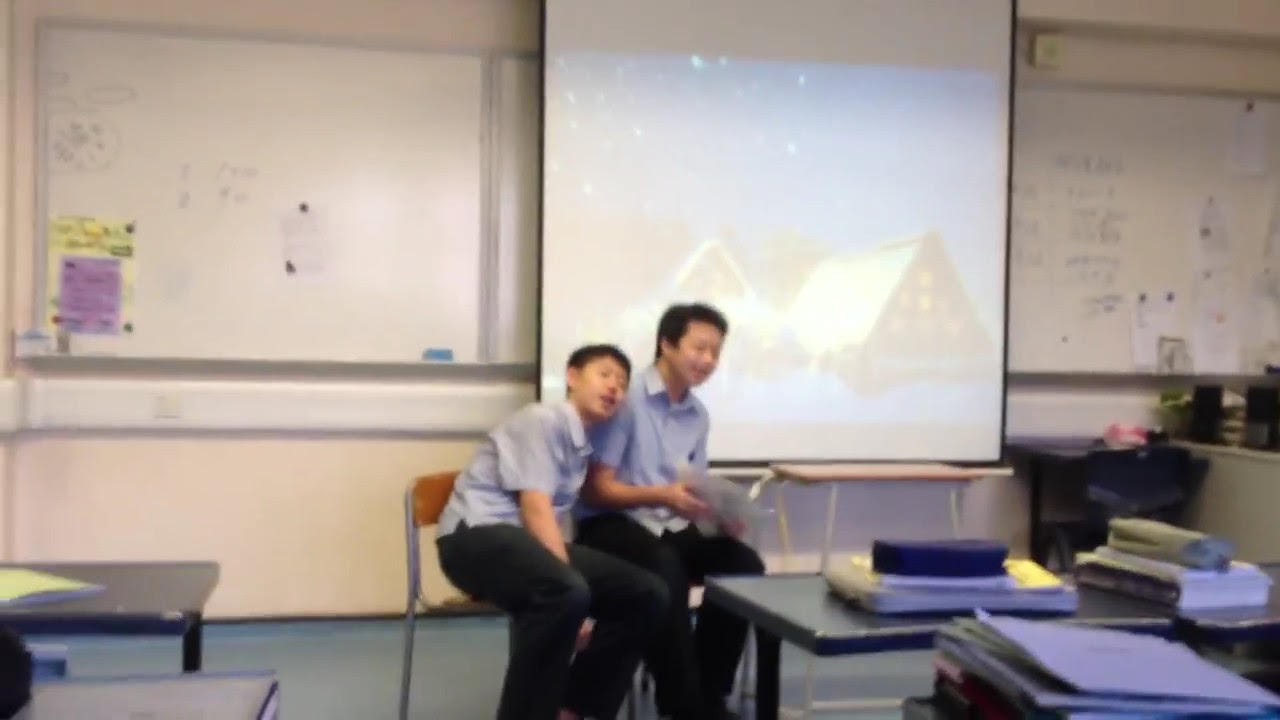In the center of this indoor classroom setting, two young Asian boys, aged between 10 and 15, sit closely together. Both boys have short dark hair and are dressed in light blue short-sleeved button-up shirts and black long pants. The boy on the left rests his head on the shoulder of the boy on the right, who appears to be holding something in his hand. 

In the background, three expansive whiteboards span the wall, adorned with various classroom formulas, letters, numbers, and signs, possibly held up with magnets. Dominating the backdrop is a large projection screen depicting an image of A-framed cottages under a starry blue sky. 

In the bottom left corner of the image, part of a desk is visible, cluttered with piles of blue folders or papers, alongside additional students' desks strewn with books and paper, reinforcing the academic ambiance of their environment.